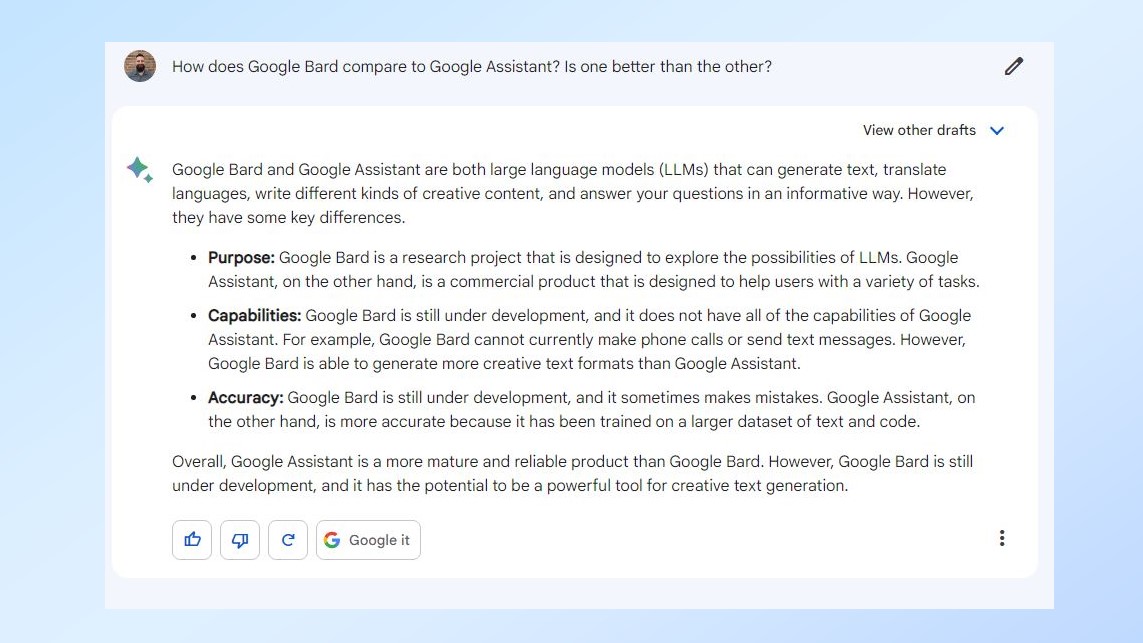The image is a screenshot of the Google Bird application, displayed on a serene pastel blue background. The focal point is the Google Bird window, which has a clean white interface framed by the pastel hue. At the top of the Google Bird page, there is a user profile image beside a question that reads, "How does Google Bird compare to Google Assistant? Is one better than the other?" Directly below this, Google Bird's detailed response is visible. The response explains: "Google Bird and Google Assistant are both large language learning models (LLMs) that can generate text, translate languages, write different kinds of creative content, and answer your questions in an informative way. However, they have some key differences." At the bottom left of the screen, user interaction options include a thumbs-up icon, a thumbs-down icon, a refresh button, and a "Google it" button for further exploration.